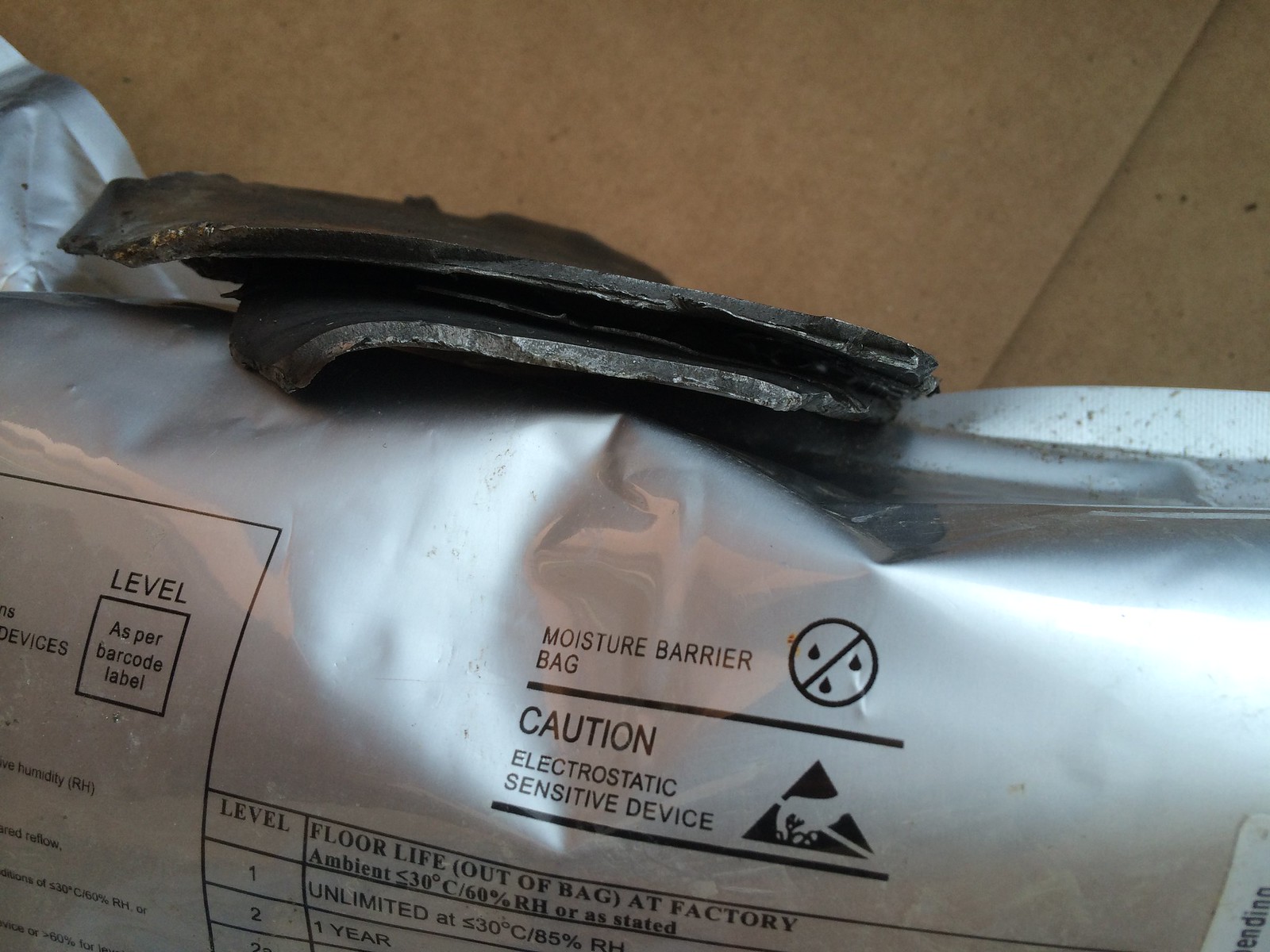This photograph captures a silver moisture barrier bag, primarily designed for storing electrostatically sensitive devices, positioned inside a brown cardboard box. The bag is distinctively marked with black text indicating "Moisture Barrier Bag" and illustrated with a no-moisture symbol—a circle with a diagonal slash through water droplets. The text on the bag also includes a caution message specifying that it contains an electrostatic-sensitive device, highlighted by a black triangle symbol with a hand inside it, signaling caution. Additionally, the bag details different levels of preservation, including information about floor life out of the bag at factory ambient conditions of 30 degrees Celsius and 60% relative humidity, with levels ranging from unlimited time for level 1 to one year for level 2. The silver bag itself appears wrinkled and somewhat cylindrical, with a couple of ambiguous black items—possibly pieces of duct tape or plastic—leaning against it. These black objects are folded over and not entirely distinct, contributing to the overall textured appearance of the setup. The scene offers a detailed view of not only the bag's functional and cautionary inscriptions but also its physical state and packing context.